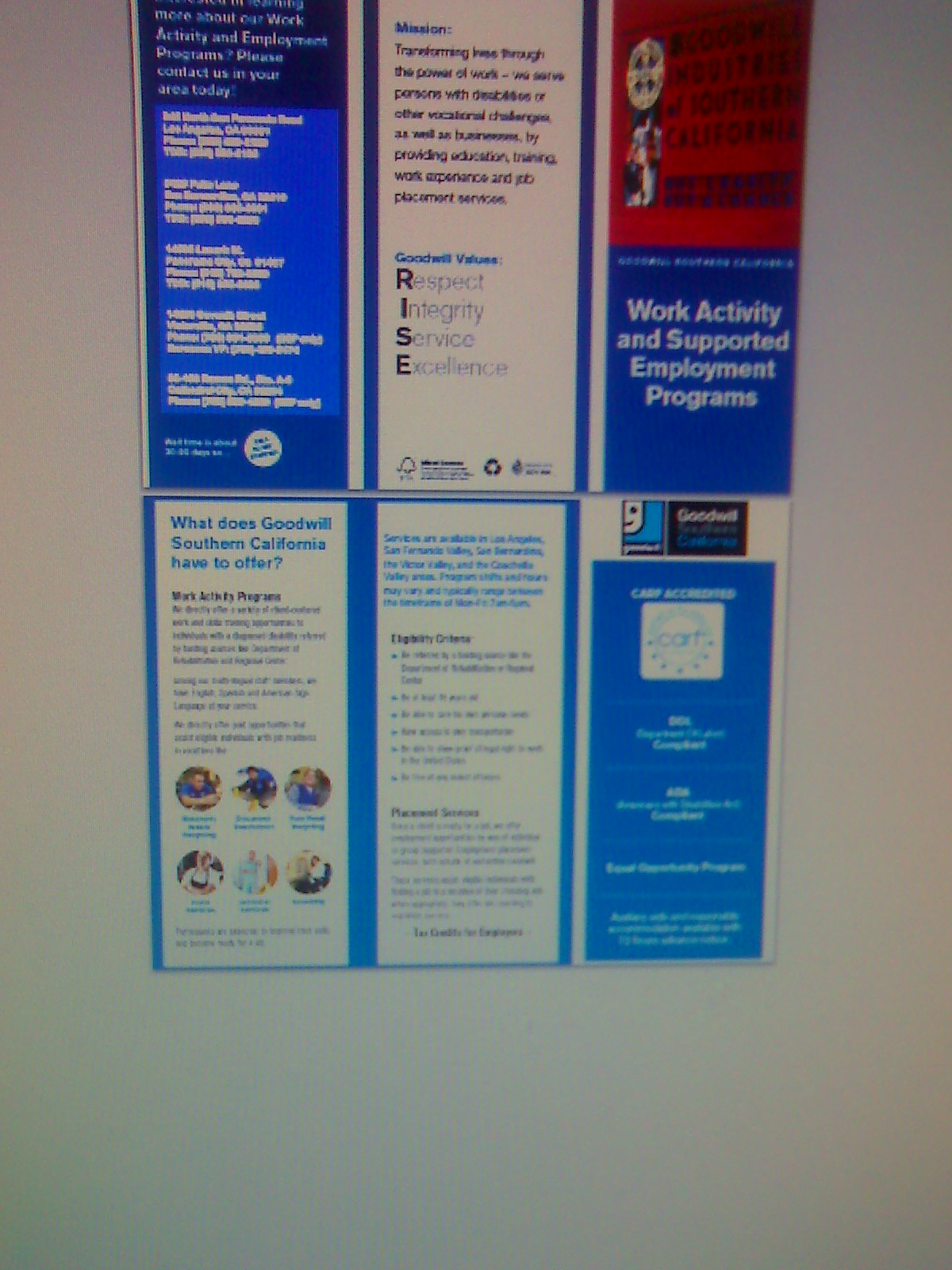This image features a flat, gray wall displaying what appears to be a poster composed of two trifold brochures positioned on top of each other. Each brochure is divided into three panels, with specific sections dedicated to different information. The top brochure includes a red upper section with a picture of a man and black letters, and a blue lower section containing white text that reads "work activity and supported employment programs." The panels have a mixture of blue and white backgrounds featuring text, although the fonts are too small to read clearly. The bottom brochure includes blue text highlighting "what this Goodwill Southern California have to offer," accompanied by the Goodwill logo in the top right corner. The middle panel on the bottom brochure provides more detailed information on a white background, while the surrounding panels display the mission statement and values of Goodwill, such as respect, integrity, service, and excellence.